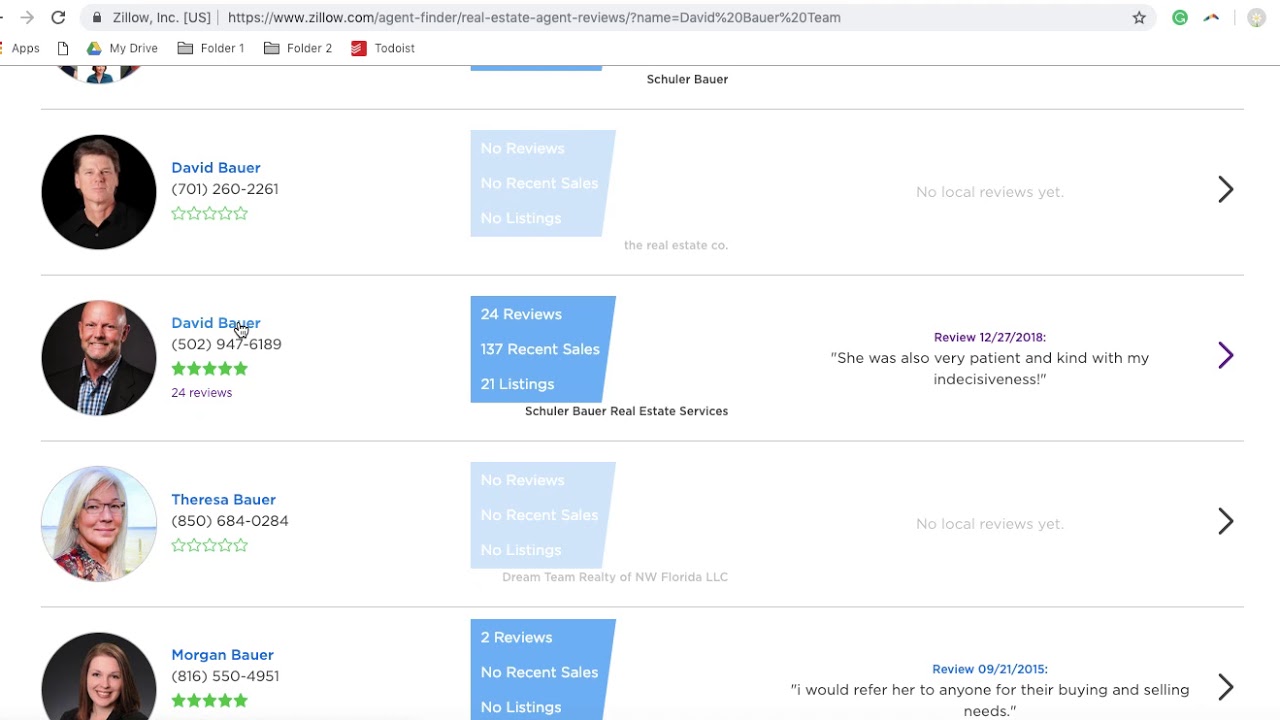In the image, there is a screenshot of a webpage on Zillow.com. At the top left of the browser is a refresh icon, followed by the URL 'Zillow.com.' To the right of the URL, there is a green icon and two additional icons. Below the address bar are various tab categories, including 'My Drive,' 'Folder,' 'Folder,' and another labeled 'Toterist.'

On the left side of the webpage, there are four profile pictures of realtors, accompanied by their contact details and reviews. The first profile is of David Bauer, featuring a phone number but no star rating listed. Directly below, another profile picture of David Bauer is shown with a phone number and a five-star rating based on 24 reviews. Following him is Teresa Bauer, who has a phone number listed but no star ratings. Lastly, Morgan Bauer is featured with a phone number and a five-star rating.

The title 'Schooler Bauer' appears to the right of the profile pictures. Below this title, there are four square shapes that alternate in color between light gray and blue. A review for David Bauer is visible, stating that "she was also very patient with my indecisiveness." For Morgan Bauer, another review says, "I would refer her to anyone for buying and selling needs." The entire webpage is set against a white background.